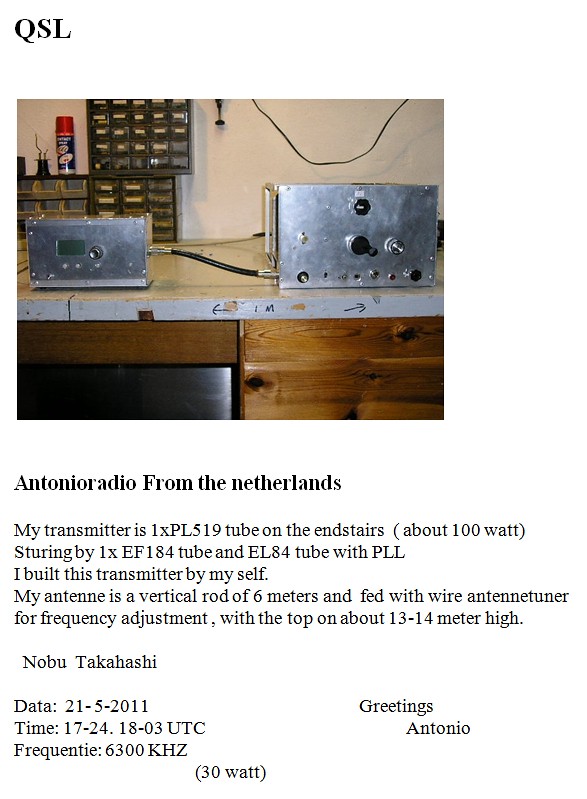The image depicts a homemade radio transmitter system resting on a workbench surface, which is a wooden table with a metal worktop. The setup features two silver cabinets linked by a black cable. The larger cabinet on the right is adorned with various dials on its surface, while the smaller cabinet on the left sports a small screen and a dial adjacent to it. A handwritten note in black ink is nearby, providing detailed specifications and context.

The text above the image reads "QSL," while text below says "Antonio Radio from the Netherlands." It includes a paragraph describing the components and construction details of the transmitter: "My transmitter is 1XPL519 tube on the end stairs, about 100 watt, steering by 1XEF184 tube and EL84 tube with PLL. I built this transmitter by myself. My antenna is a vertical rod of six meters and fed with wire antenna tuner for frequency adjustment with the top on about 13 to 14 meter high." Below, the text continues with Nobu Takahashi’s name and date: 21.5.2011, time: 17.24.18.03 UTC, frequency: 63.0.0.KHZ, and a greeting from Antonio along with "30 watt" noted at the bottom center.

The transmitter, intricately built with detailed documentation, reflects the dedication and craftsmanship of its maker, showcasing an impressive endeavor in radio technology.